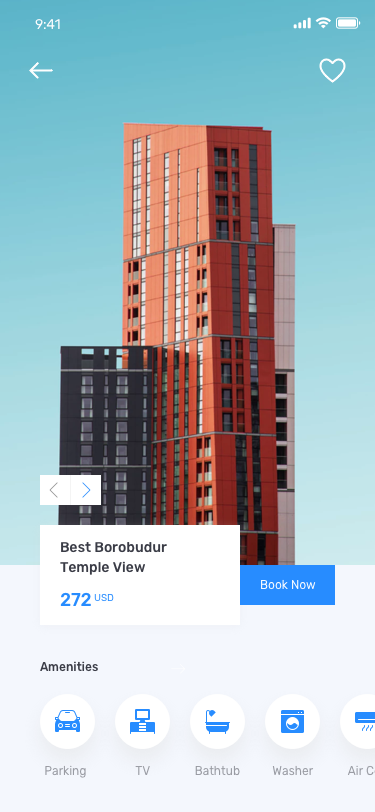This screenshot, captured from a mobile device, showcases an open app with an elongated, rectangular aspect ratio indicative of smartphones. The status bar at the top of the screen displays full battery life, strong cell signal, and active Wi-Fi connection, along with the time reading 9:41 (AM or PM is unspecified).

The background of the app features a light blue sky with a striking architectural complex comprised of three interconnected buildings. The central and tallest structure, resembling a vertically stood Jenga piece, is a burnt orange color. Connected to it are two other buildings: a shorter black building on the left and a slightly shorter white building on the right.

In the lower part of the screenshot, there is a prominent box displaying the text "Best Borobudur Temple View 272 USD book now," suggesting that rooms with this view are available for booking at a cost of 272 USD. At the bottom of the screen, a series of icons are visible, likely representing various amenities that can be selected when reserving a room in this unique architectural setup.